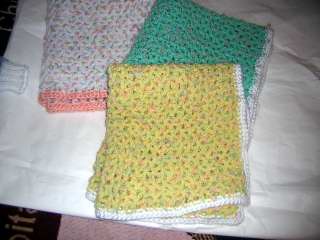This indoor photograph showcases three small, handmade crocheted items, likely blankets or dishcloths, meticulously folded and displayed on top of a thick, folded white fabric. The piece nearest to the viewer is a pale yellow blanket with a white border, featuring subtle hints of green and pink yarn woven into it. Beneath this, a bold teal-colored piece with a white edge is partially visible. To the left and slightly underneath these is a white variegated blanket adorned with pastel colors like pink and yellow, bordered by a peachy pink edge. The blankets are neatly stacked, and there is a small section of text in light pink towards the lower left corner of the image.